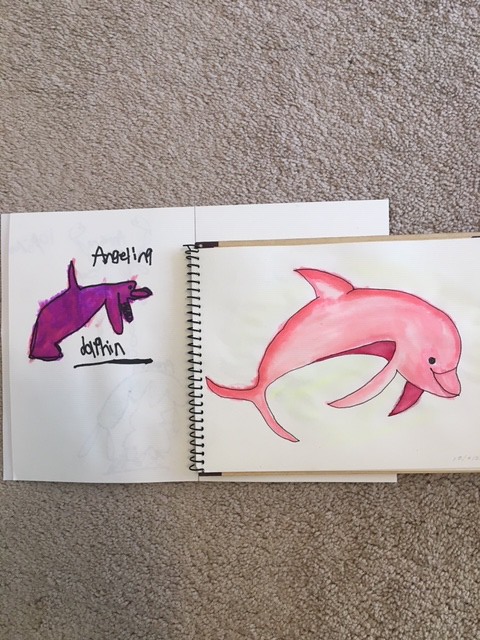The image features a sketchbook with a spiral binding resting on a tan carpet, surrounded by additional sheets of drawing paper. On the open page of the sketchbook, there's an intricately shaded, coral pink dolphin, gracefully arched as though leaping out of the waves, with a cheerful expression. Adjacent to this, another sheet partially extends from the sketchbook, displaying a less skillfully drawn purple dolphin. Above this purple dolphin, the name "Angelina" is written, and "dolphin" is inscribed below it. The combination of these drawings suggests that while one artist has achieved a higher level of proficiency with their pink dolphin, another, likely indicated by the name "Angelina," is still in the early stages of developing their drawing skills.